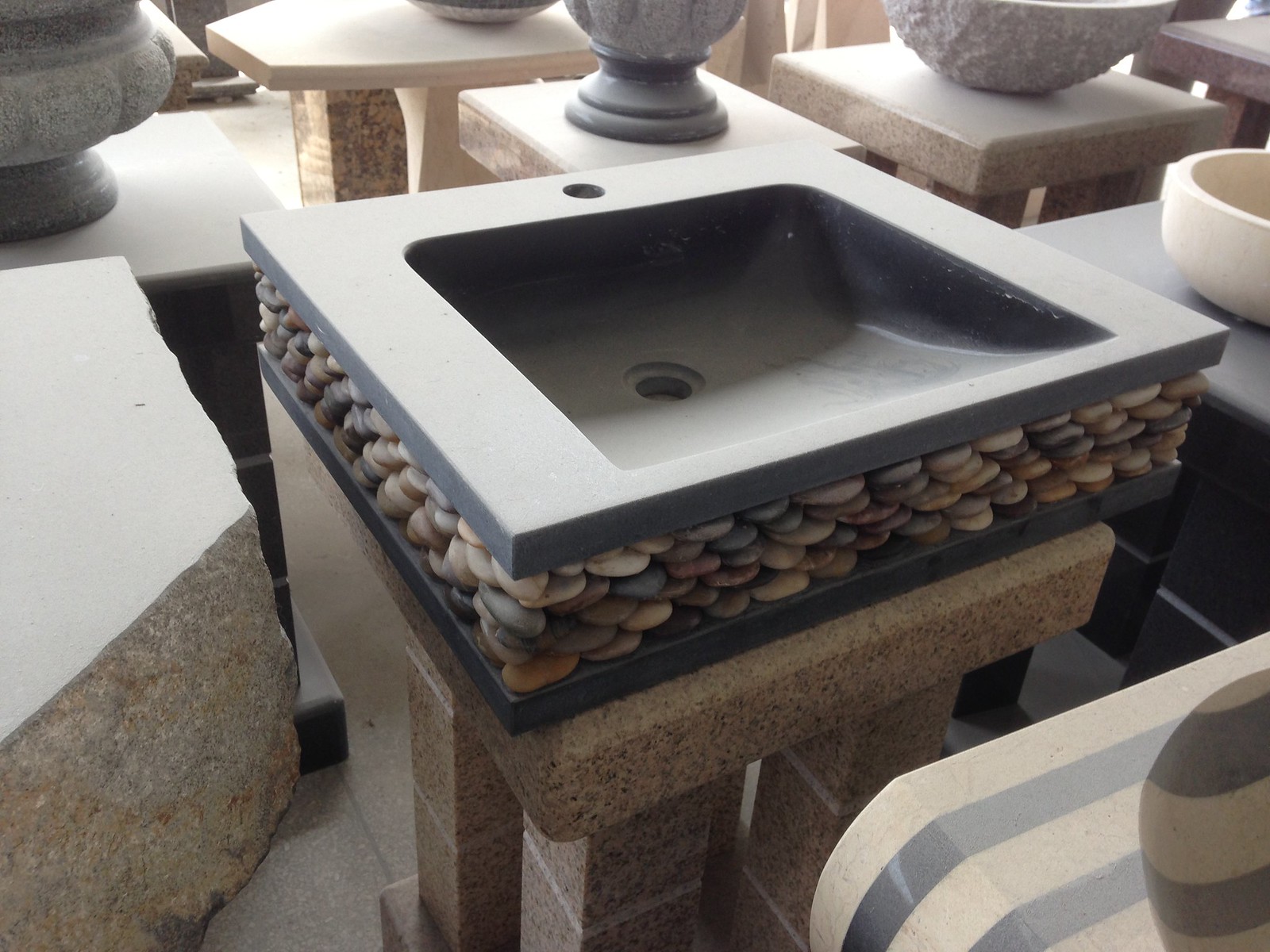This image captures an eclectic assortment of stone and ceramic objects densely displayed in a confined space. The room appears overcrowded, making it challenging to navigate between the items. Various tables of differing shapes, sizes, and heights fill the room, with a predominance of square tables interspersed with a few uniquely shaped ones, including five-sided tables. 

On the left, a significant stone piece stands out with its depth of approximately two feet and a remarkably smooth surface. The centerpiece is an intricately designed sink. This sink features a one-inch thick flat stone top and a stone basin with a matching stone bottom. The edges of the sink extend to form a shallow basin, complete with a hole for draining and another for a faucet. The base of the sink is cleverly constructed with smooth river stones stacked together, creating a visually appealing "stone sandwich" effect.

Additionally, the tables are adorned with various bowls. These include small, white bowls alongside a rougher, stone bowl with varying degrees of polish, adding to the textural diversity of the display.